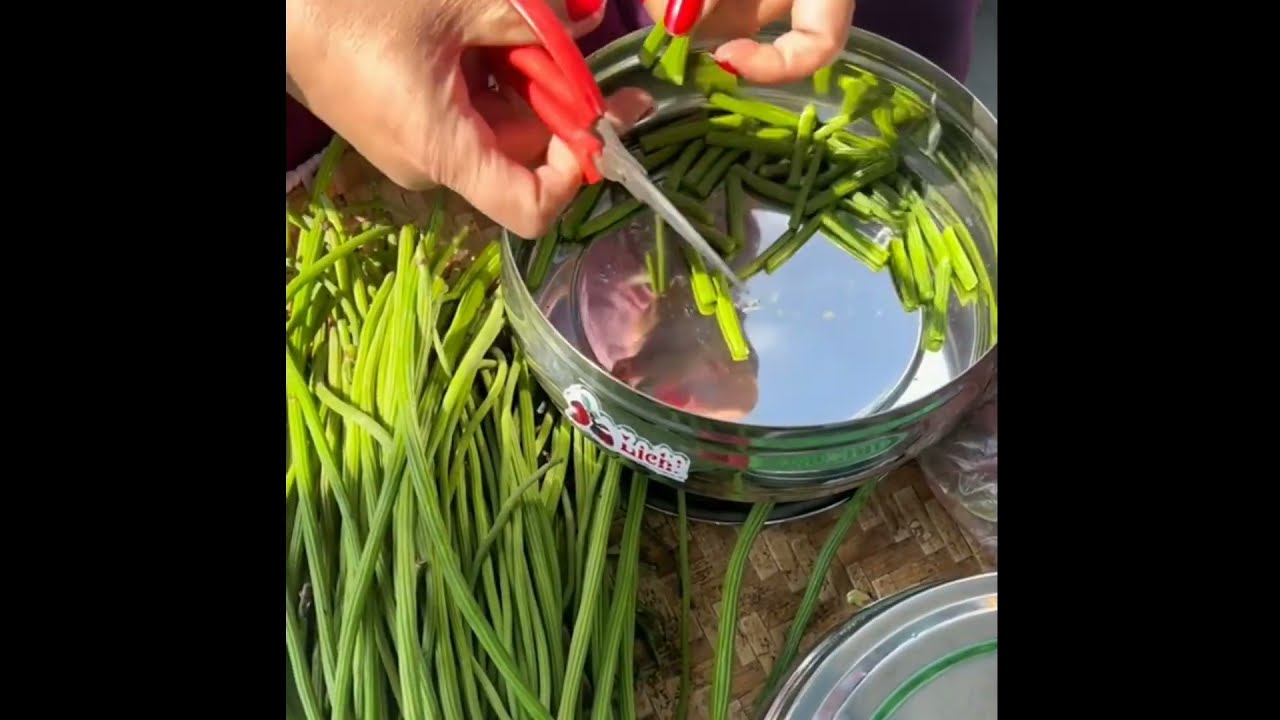This detailed photograph depicts a table setting taken from above, featuring a pair of hands adorned with red nail polish, engaged in preparing green vegetables with a pair of red-handled scissors. The vegetables, identified as string beans due to their thin and long appearance, are being carefully trimmed and placed into a silver container, which possibly contains water for washing. The image has a mix of sunlight and shade, creating a dynamic lighting effect. To the left and right sides of the frame, there are black vertical strips. Additionally, white plates are present on the table. The scene possibly takes place outside, adding a natural lighting element to the composition. The woman's methodical work with the red scissors suggests she is diligently cleaning and preparing the string beans as part of a meticulous cooking process.